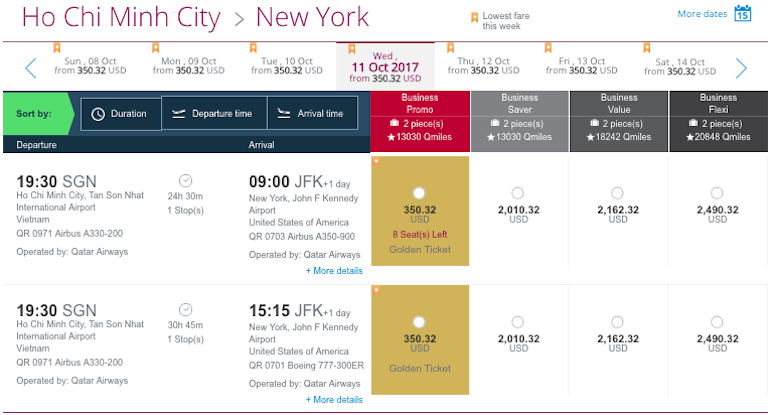The image appears to be a detailed scheduling interface or travel itinerary with various sections and colors indicating different types of information. Here's the descriptive caption:

At the top of the image, the text "Ho Chi Minh City" is displayed in pink, accompanied by a grayish-blue arrow pointing to the right, followed by the text "New York," also in pink. Below this, a small bookmark icon is present next to some illegible text. 

Further down, blue-colored text lists additional dates, situated next to a blue calendar icon. A reddish horizontal line divides this section from the rest.

On the left side, a blue arrow points to the left, and on the right side, a blue arrow points to the right. Between these arrows, column-like structures resembling bookmarks run vertically down the image, each accompanied by text, although the inscriptions are too small to read. 

In the central area, a bookmark-like element with a gray background displays the date "11 OCT 2017," with additional information below it.

Towards the bottom, a blue rectangle with a green arrow pointing to the right contains the label "sort by." Below this, three darker blue rectangles are present. The first rectangle, marked with a clock icon, indicates "duration;" the second, showing an ascending airplane icon, reads "departure time;" and the third, with a descending airplane icon, states "arrival time." This is followed by text "departure and arrival."

Below this section, a red rectangle with unreadable text is followed by a series of gray rectangles varying in shade from light to dark, all containing text that is too small to decipher. 

Underneath, the time "19:30" is labeled with "SGN" and followed by an abundance of small, illegible text. This pattern repeats: the time "19:30 SGN" appears again, followed by more small text.

Two circles, potentially resembling clock faces, are positioned on the left. To the right, the time "09:00" labeled "JFK" appears, paired with more small text. Further down, "15:15 JFK" is similarly accompanied by text that remains difficult to read.

At the bottom, two dark yellow rectangles contain additional small text, and six circles are organized into two rows of three. Each circle displays a number with a word beneath it.